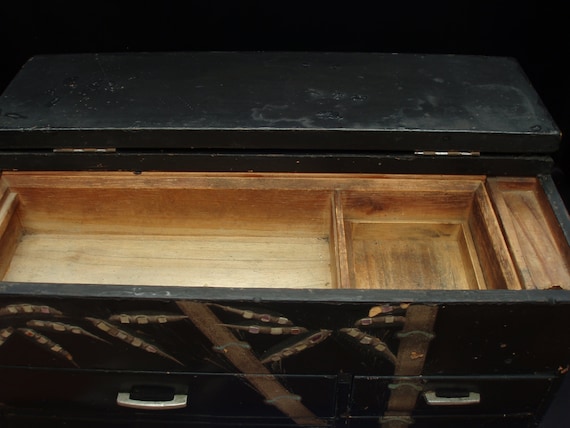This indoor photograph captures a close-up view of an open desk drawer set against a dark brown and light brown wood interior, which appears unfinished and heavily worn with black spots and stains. The exterior of the drawer is made of dark black wood, featuring two metallic handles on either side, positioned left and right. The drawer also has decorative floral and tree branch motifs, painted in black with scattered branches, lending an artistic touch to its design. The drawer is centrally located in the image, spanning from left to right, with its open top revealing the upper surface of the cabinet, which shares the same black wood color.

Above the main drawer, the top section of the cabinet or desk is visible, showing an open lid section that flips backward and is divided into three areas: a large compartment on the left, a medium-sized one on the right, and a tiny section on the far right. This open lid reveals more internal storage spaces that can house various items. The overall look of the photograph clearly emphasizes the age and wear of the furniture piece, with significant detailing in both the wood's texture and the painted decorations. There is no text present in the image.